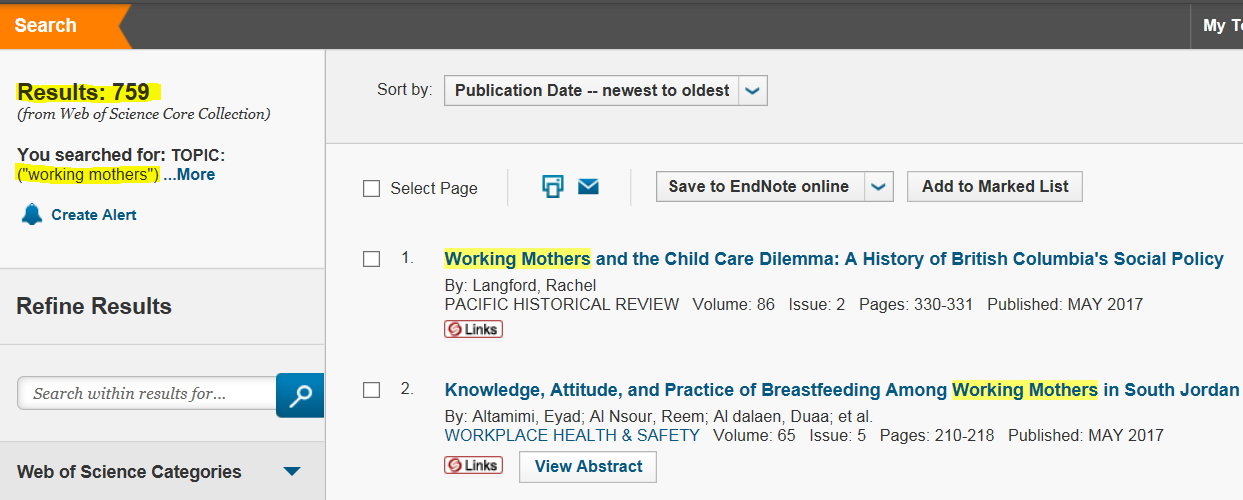The image showcases a user interface from a research database. 

In the top left corner, a small orange banner displays the word "Search," immediately followed by a black banner stretching across the width of the interface.

Beneath these banners, the text "Results: 759" is prominently featured. In parentheses, it specifies that these results are sourced from the "Web of Science Core Collection." Below this, the phrase "You searched for: Topic: Working Mothers" is highlighted in yellow.

Adjacent to this, there is an option labeled "More..." which expands to provide additional information when clicked. Below, a blue button labeled "Create Alert" accompanied by a bell icon allows users to set up notifications.

Further down, the section titled "Refine Results" includes a search bar with the placeholder text "Search within results for..." and a blue magnifying glass icon. Users can enter keywords here and click the magnifying glass to further filter their search results.

Following this, the "Web of Science Categories" section displays a blue arrow that, when clicked, drops down to reveal more detailed categories.

In the main body of the image, a list of results is shown. The first result is titled "Working Mothers," and the second result is "Knowledge, Attitude, and Practice of Breastfeeding Among Working Mothers in South Jordan."